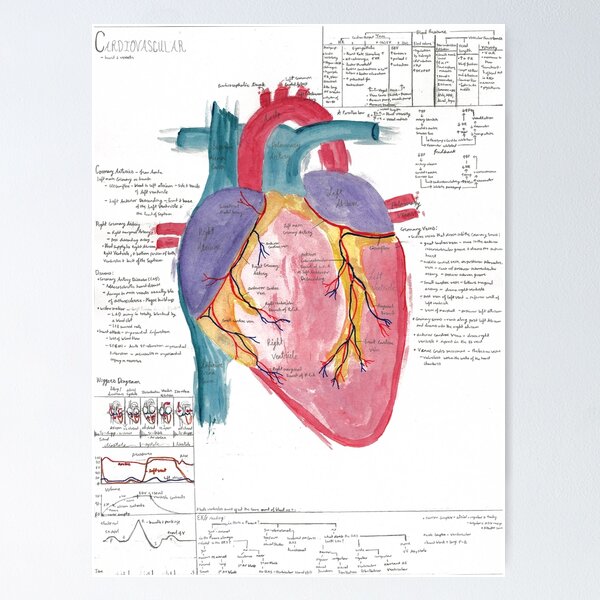The image features a meticulously hand-drawn and labeled diagram of the human heart, created using a combination of watercolor or pen and ink on heavy or watercolor paper. Dominating the center, the heart is illustrated in vivid sections of red, teal, purple, yellow, blue, and pink, each color likely corresponding to different anatomical features and functions. At the top left corner, the word "cardiovascular" is prominently displayed, indicating the focus of the diagram. Surrounding the heart are numerous detailed handwritten annotations and charts, meticulously outlining and explaining the various parts and mechanisms of the cardiovascular system. Although the text is too small to decipher in full, the careful craftsmanship and in-depth commentary suggest this is a student's school assignment aimed at capturing the complexity of the heart and its functions. The entire drawing is set against a clean, white background with the paper itself framed by a light grey backdrop.